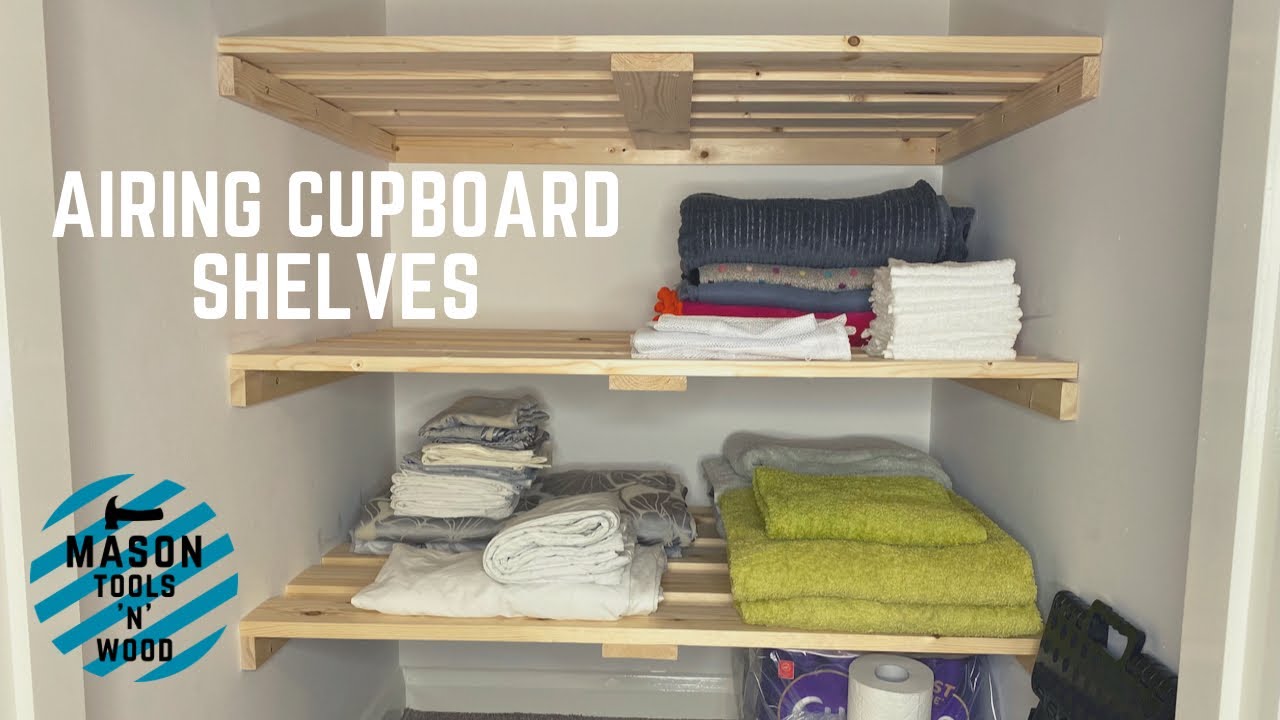The image depicts an organized pantry or large closet featuring three neatly installed wooden shelves, making for a practical advertisement. The top shelf, made from what appears to be simple wood, is empty. The middle shelf holds folded white hand towels and some bath towels in varying colors, including blue. The bottom shelf is occupied by neatly arranged white and gray sheets alongside light green towels. Below the bottom shelf, on the ground, there are rolls of toilet paper and a step stool. The shelves, which resemble wooden pallets, are carefully mounted against a white wall and are each about a foot or two deep, separated by approximately a foot and a half of space. To the upper left, in white text, the image is branded with "Airing Cupboard Shelves." At the bottom left, a light blue circle with diagonal stripes showcases the logo for "Mason Tools and Wood" in black text, complete with a hammer icon.